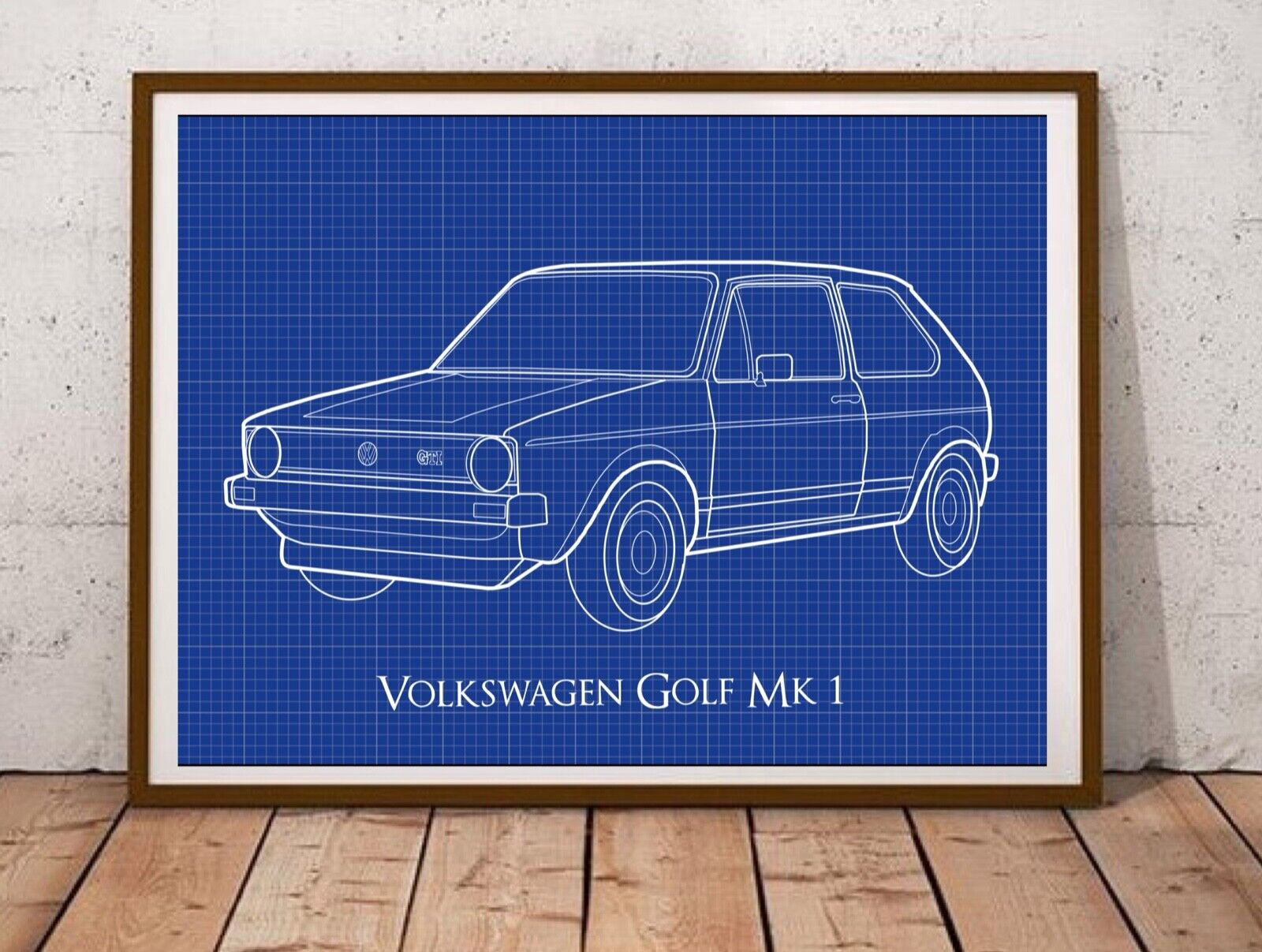The image showcases a detailed blueprint of a Volkswagen Golf Mk1, drawn in white ink on a blue, graph-like paper, highlighting a meticulous representation of the car's structure. This artwork, framed by a wooden border and featuring a white margin, lies on top of a wooden plank floor. The background consists of a cement-gray wall, imperfect with small holes and marks, adding a raw, industrial feel to the scene. The primary focus is the precise, white ink drawing of the Volkswagen Golf Mk1, contrasting vividly against the blue grid paper, capturing the essence of engineering and design.